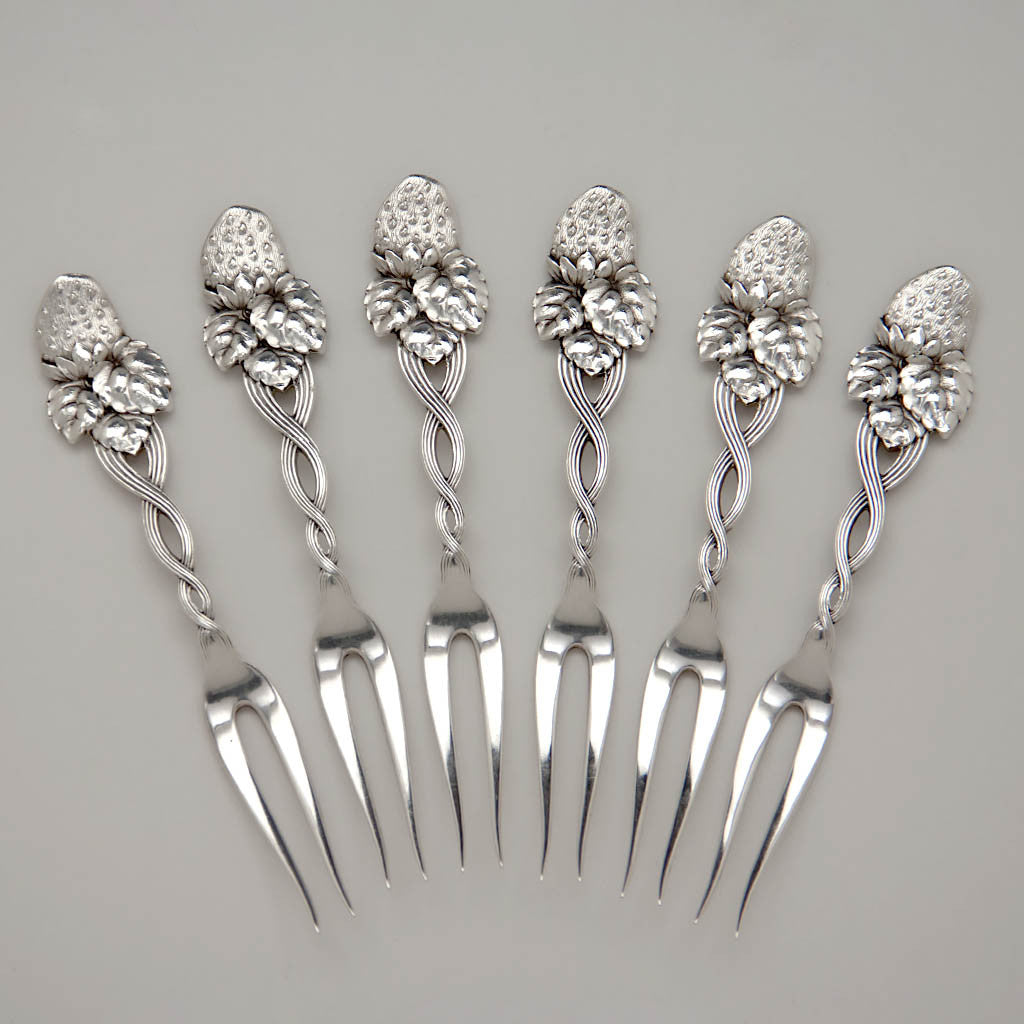The image depicts six exquisitely crafted, silver specialty forks, each featuring two prongs. The handles are intricately twisted in a braided pattern, creating a series of gaps. At the top of each handle, there is a meticulously carved set of strawberry leaves and a single strawberry, complete with detailed seeds, highlighting the hand-carved craftsmanship and distinctiveness of each fork. The forks, polished to a high shine, are arranged in a downward-facing, semicircular formation on a gray background, likely a table. This setting evokes an air of sophistication, reminiscent of high-end dining experiences in exclusive, expensive restaurants. The professional quality of the photograph enhances the elegance and allure of these luxury dining implements.